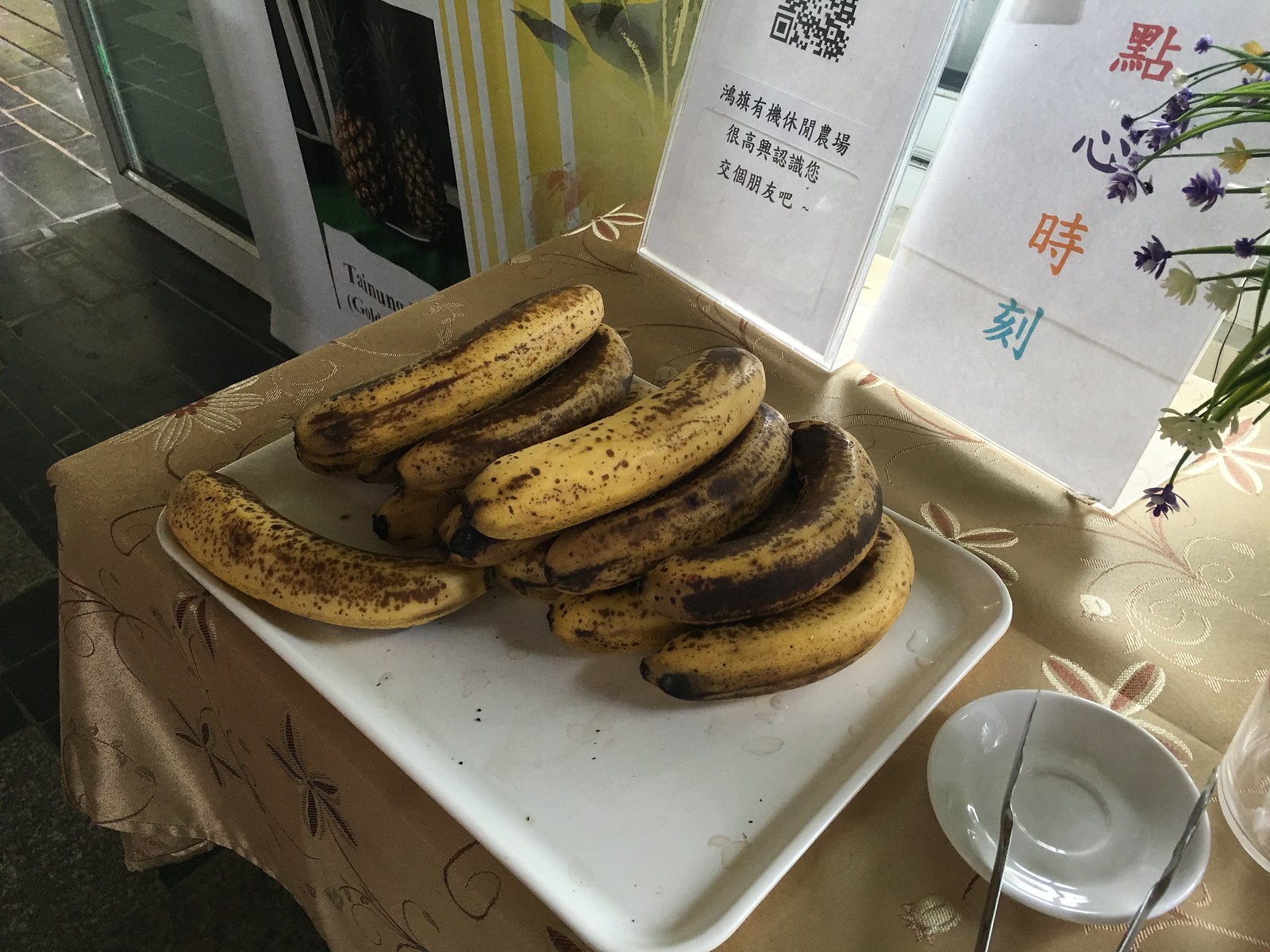This colour photograph presents a first-person perspective of a breakfast buffet offering in what appears to be a hotel lobby or meeting room. The focal point is a rectangular white tray with curved corners, laden with a large bunch of overripe bananas. The bananas exhibit a heavily spotted yellow skin, some with black spots and others almost entirely black, displaying telltale signs of extreme ripeness. One banana is positioned at a 90-degree angle to the rest. To the right of the tray, a white ceramic saucer holds a pair of silver tongs, reinforcing the buffet setting.

The tray rests on a tan, shiny, and silky tablecloth adorned with intermittently embroidered white floral patterns. Behind the tray are two acrylic sign holders with upward-leaning signs, featuring traditional Japanese characters and a QR code. The room's ambiance includes a golden yellow wall with white vertical stripes and a grey block-patterned floor. Light streams into the room from a door in the upper left corner and a window behind the bananas, enhancing the overall warmth of the setting. To the left of the tray is a partially visible door, suggesting a likely entrance or exit. The upper right-hand corner of the image also captures a glimpse of a plant with small leaves and bluish buds or flowers.